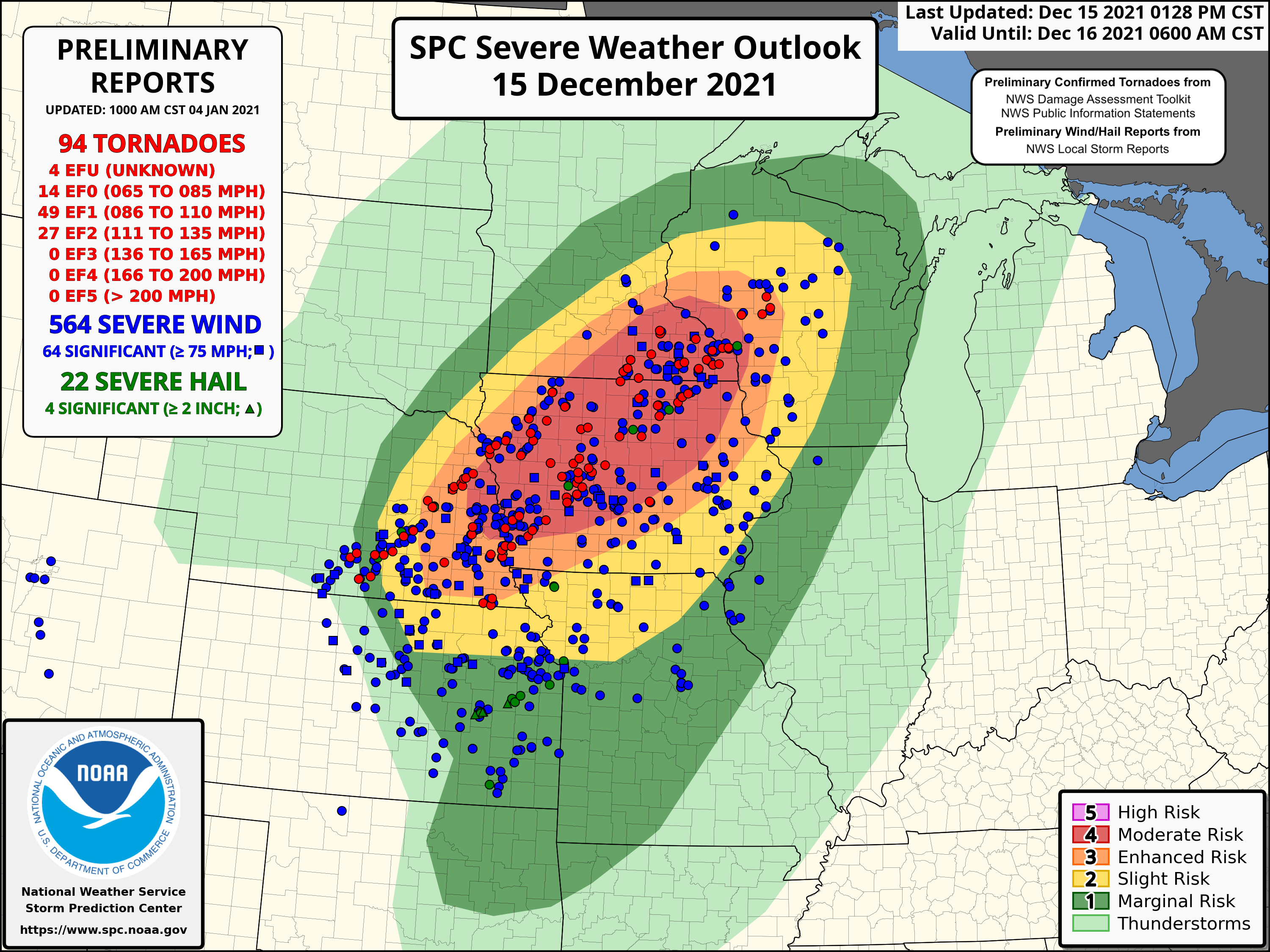This image is a detailed map titled "SPC Severe Weather Outlook, December 15, 2021," from NOAA's National Weather Service Storm Prediction Center (SPC). It focuses on the upper Midwest region, specifically depicting areas in Illinois, Indiana, Michigan, and Wisconsin. The map is marked with several color-coded layers indicating different levels of severe weather risk: green for marginal risk, yellow for slight risk, orange for enhanced risk, and pink for high risk. A lighter green area is also shown, denoting thunderstorm activity.

In addition, the map features pins and dots representing weather reports. Blue dots highlight areas of severe wind activity. Preliminary data included in the graphic lists 94 tornadoes reported on that day, with a breakdown of their intensity: 4 EF-U (unknown intensity), 14 EF-0, 49 EF-1, and 27 EF-2. The map also notes 564 severe wind reports—64 of which were significant—and 22 severe hail incidents. There is a small box on the map specifying these statistics, providing a comprehensive view of the severe weather occurrences of the day.